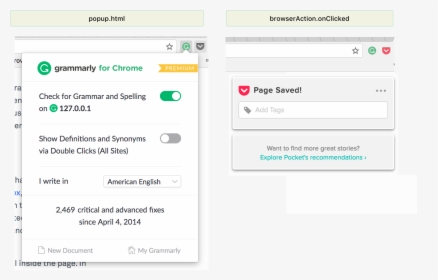The image depicts a pop-up interface of the Grammarly browser extension on a computer screen. In the top right-hand corner of the screen, there is a green circle icon featuring a white arrow that curves counterclockwise, indicating the Grammarly extension is active. Adjacent to this icon, text reads "Grammarly for Chrome," accompanied by a yellow premium ribbon, signifying additional features available for paid subscribers.

Within the pop-up, several settings and options are visible. The primary option shows that the Grammarly extension is turned on, denoted by the phrase "Check for grammar and spelling on Grammarly" with a switch indicating the feature is active. Beneath this, there is another setting labeled "Show definitions and synonyms via double clicks," which is turned off.

Further down, the language preference is displayed, indicating that the user writes in "American English." Under the language setting, statistics reveal that since April 4th, 2014, the user has made 2,069 critical and advanced corrections with the assistance of Grammarly.

To the right of this Grammarly pop-up, there is a smaller, additional notification stating "Page saved." This secondary pop-up is distinguished by its red color and contains a white downward-pointing arrow, suggesting another functionality likely related to saving progress or settings on the webpage.